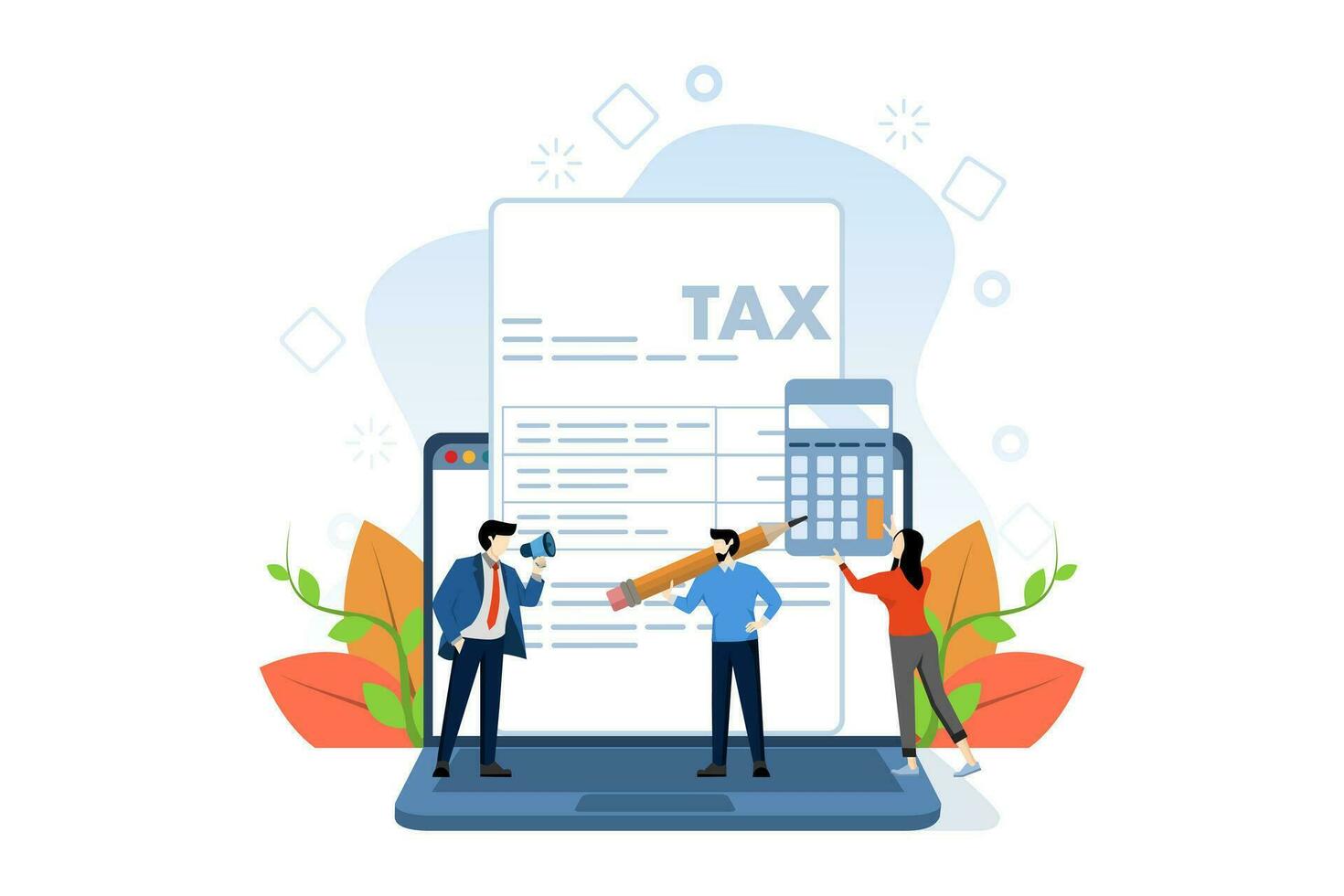This detailed digital image showcases an animated, cartoon-style scene that appears to be an advertisement for tax paperwork. Central to the scene is an open blue laptop with a white screen featuring blue lines and a small red and yellow dot. In front of the screen, a white document with mock writing and the prominently displayed word "TAX" in blue letters stands vertically. 

Standing on the laptop's keyboard are three cartoon characters. The first character, on the right, wears a blue suit with a white shirt, red tie, and blue pants, holding a megaphone to his mouth. The middle character, wearing a blue shirt and jeans, hoists a giant pencil over his shoulder. The third character, on the left, has long black hair and wears a red shirt with gray pants, holding an oversized calculator. 

The background features various light blue designs, including squares, circles, and star-like shapes. Additionally, the image includes two leaves—one orange and the other salmon pink—connected by a green vine, adding a touch of natural elements to the composition.